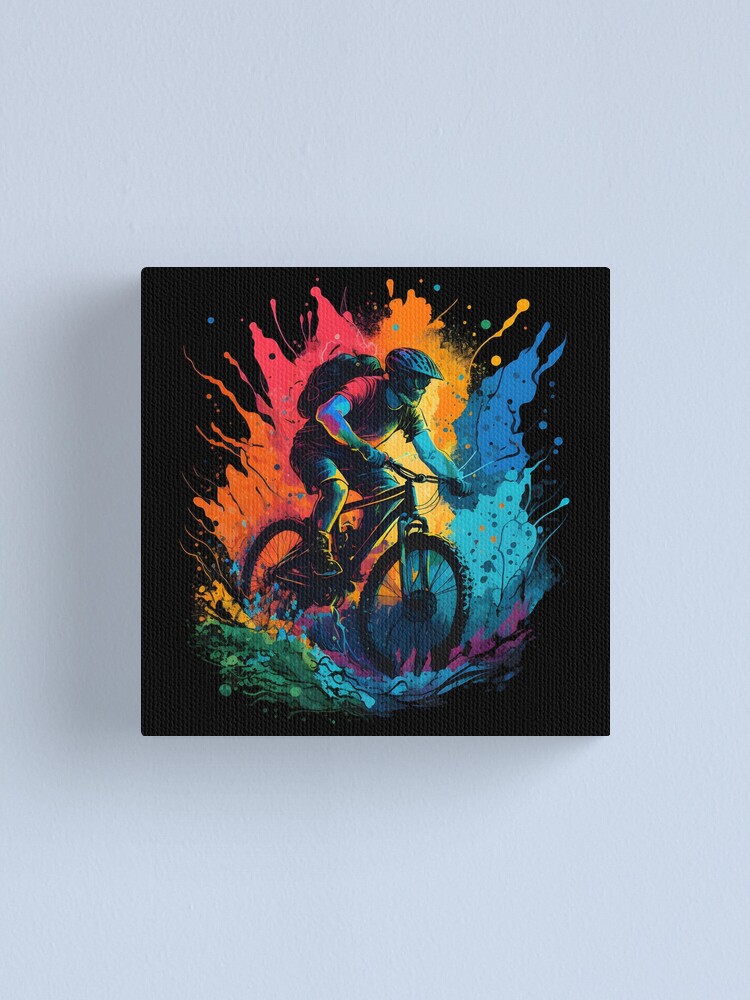The picture shows a dynamic and colorful painting hanging on a light blue wall. The painting features a black background adorned with an explosion of vibrant, splattered colors. Blues, greens, and purples dominate the bottom section, transitioning to an array of blues, turquoises, and pinks on the right side. Bright splashes of orange, yellow, and pink further animate the scene, creating an energetic atmosphere.

At the center of this vibrant chaos is the silhouette of a man on a mountain bike, depicted with striking detail. He's equipped with a helmet and a face mask, wearing a layered outfit that includes a red shirt over a long-sleeve white shirt, shorts, and boots. His arms appear blue and his legs yellow with blue highlights, contributing to the multicolored aesthetic. A black backpack is strapped to his back.

The man’s bike boasts large, prominent tires, further emphasizing the ruggedness of the scene. The entire composition bursts with energy, making it appear as though the man is riding through a whirlwind of paint, with colors exploding around him like flames, suggesting a thrilling and intense ride through a vividly imagined landscape.